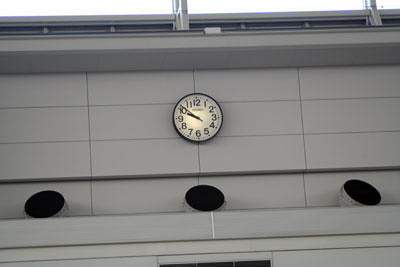This photograph captures an outdoor clock affixed to the side of a gray building, possibly a courthouse or government establishment. The building is constructed from smooth, rectangular bricks and features detailed architectural elements along its upper section. Situated below the clock are three metallic pipes, resembling exhaust pipes. The clock itself is of a standard round design, with a white face, black numerals, and three distinct hands: a long minute hand, a short hour hand, and a red second hand. The clock is softly illuminated, imbuing it with a gentle glow that accentuates its presence against the building facade.